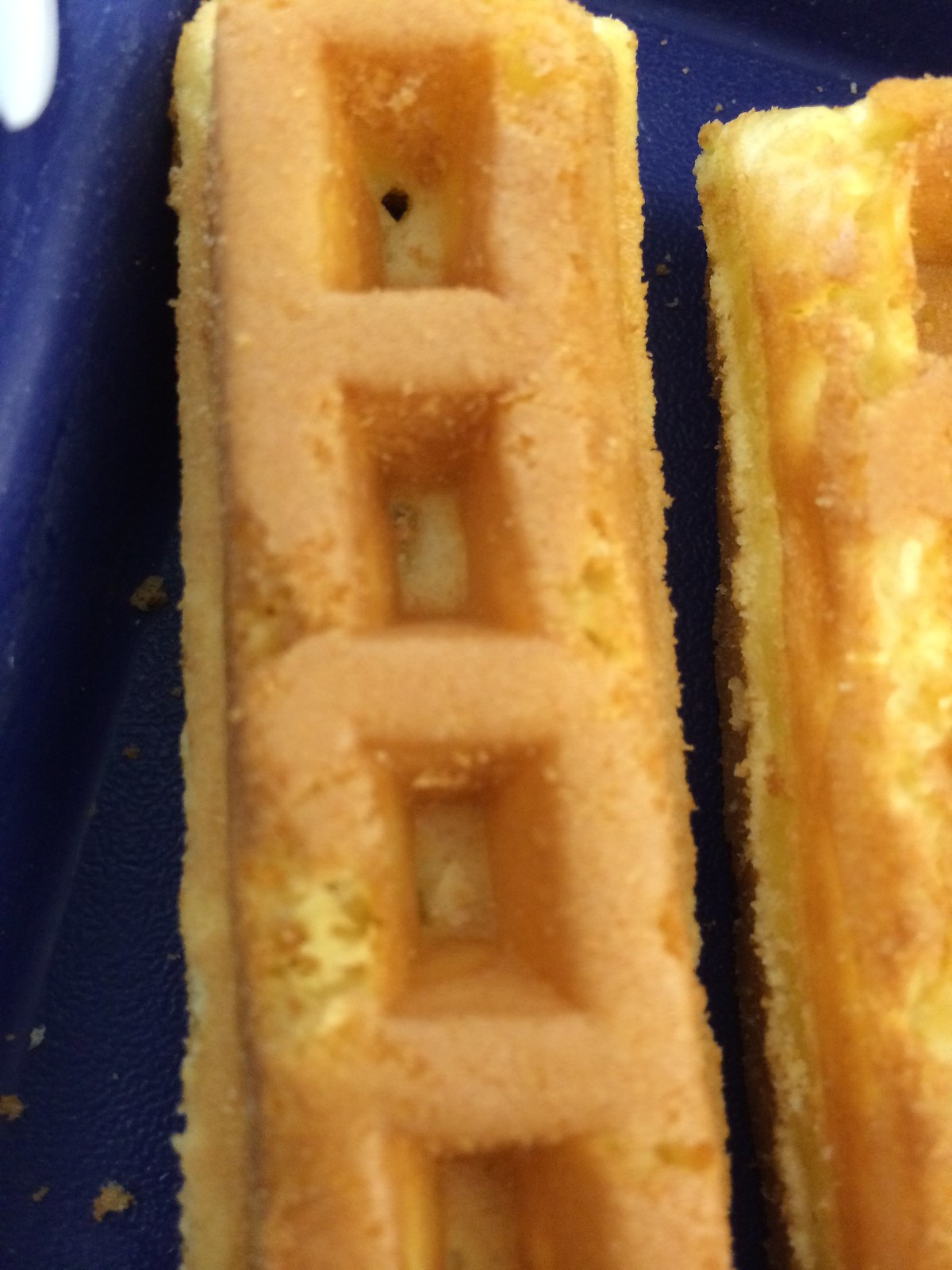The color photograph in portrait mode features a close-up of two strips of square waffles set against a rich navy blue background, likely a fabric or tray. One narrow strip with four deeply indented waffle squares is prominently displayed, giving it a cave-like appearance inside. The waffle on the right has a golden-brown toasted surface with a hint of a light yellow crust, transitioning to a darker brown towards the edges. The rectangular waffles run diagonally up and down the frame. The edges are slightly crumbly, with a few crumbs scattered in the bottom left corner of the image. In the upper left corner, there's a small white reflection adding a subtle detail. The photograph captures the texture and color variations of the waffles, showcasing both their golden-brown toasty parts and their lighter yellow central sections.